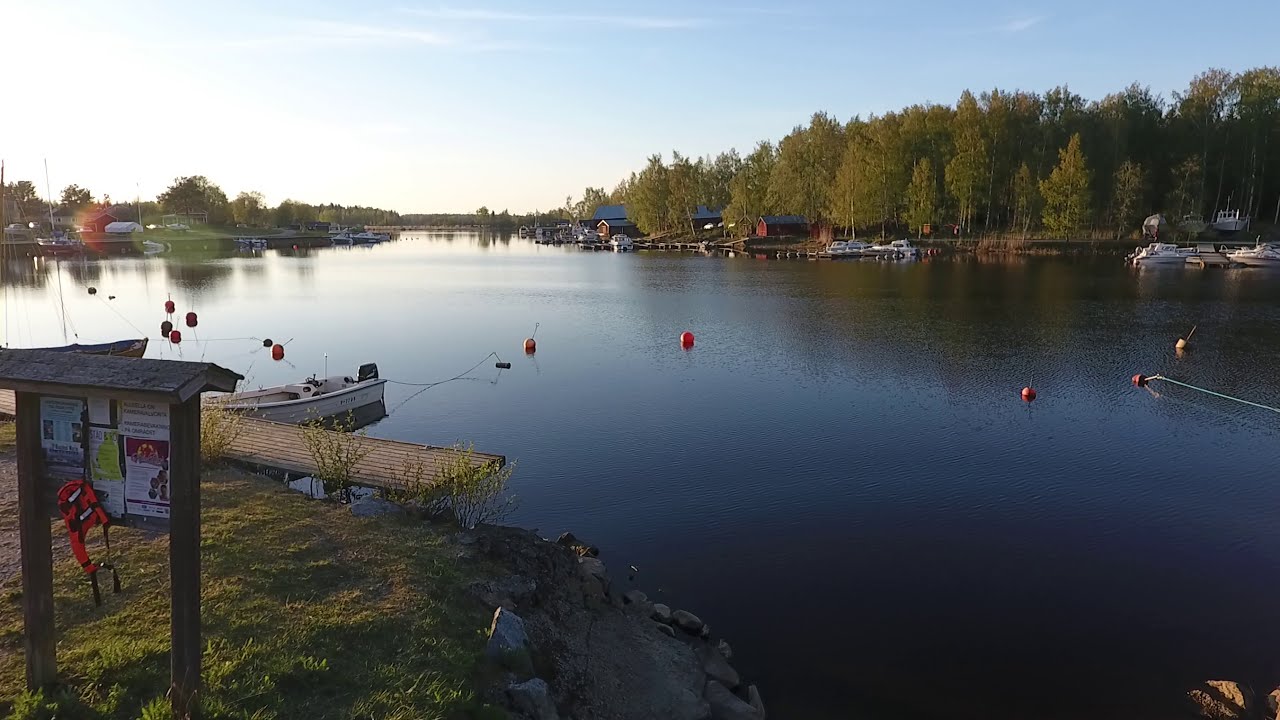The photograph captures a serene recreational lake scene during daylight, possibly close to sunset, enveloped in lush natural surroundings. In the lower left foreground, there's a grassy patch featuring a bulletin board adorned with numerous flyers and a conspicuous orange high-visibility belt, topped by a small arched roof. Beyond this, a dock accommodates a boat, while several orange buoys float calmly on the still water, creating a tranquil ambiance.

Across the lake, multiple motorboats, some with cabins and some without, are moored along wooden pontoons and platforms. The far side of the lake on the left and right reveals a mix of buildings, including what appears to be cabins and barns, creating a picturesque shoreline interspersed with grassy areas and more boats.

Vibrant reflections of the surrounding lush green trees dance on the water’s surface, enhancing the scene's natural beauty. The sky above is a brilliant blue with hints of white clouds, basking the entire area in natural light, creating a richly detailed image with varying colors from the vegetation and structures. Overall, the image offers a clear, vivid snapshot of a peaceful lakeside retreat.